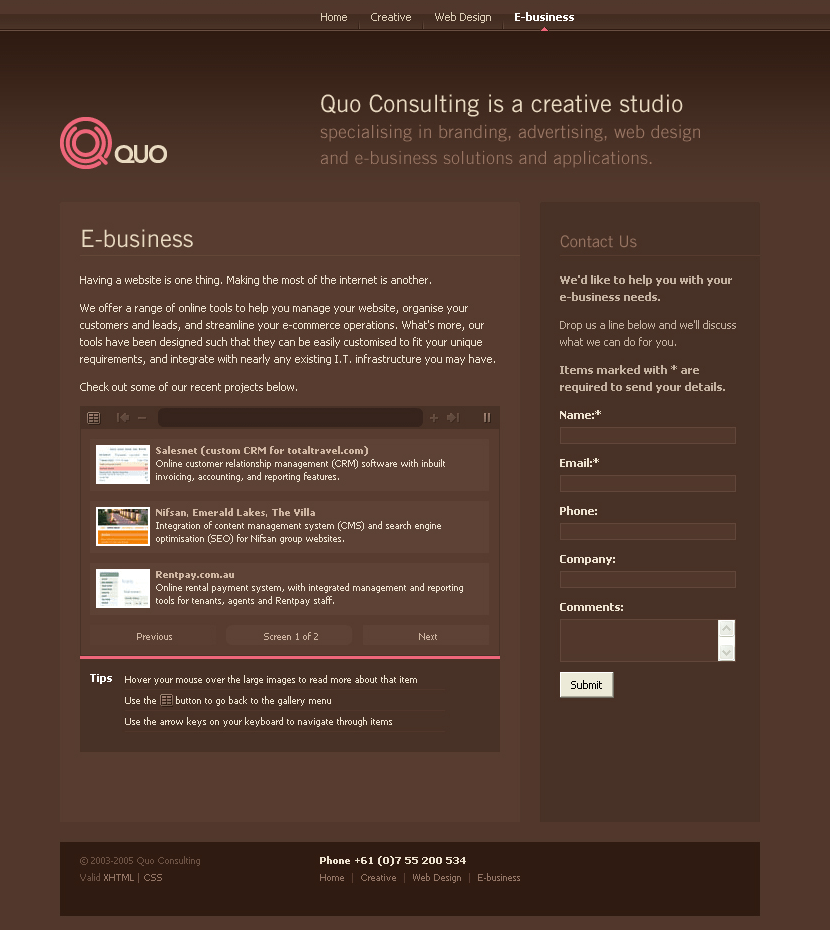**Screenshot Description of a Website's E-Business Page**

The screenshot captures a website interface dominated by a dark color palette, ranging from black to dark brown. At the top, a similar-colored banner runs across, housing four centered navigation tabs: "Home," "Creative," "Web Design," and "E-Business." The "E-Business" tab is selected, distinguished by its white font and a red arrow beneath it.

Beneath the banner, the main content area starts on the left with a small icon labeled "QOQUO," followed by the text "QO Consulting as a Creative Studio." In a less bold font below, the description reads: "Specializing in Branding, Advertising, Web Design, and E-Business Solutions and Applications."

Further down, a faint, wide box contains indented text starting with the heading "E-Business." The subsequent smaller font text reads, "Having a website is one thing, making the most of the internet is another." This is followed by another paragraph detailing the business's offerings: "We offer a range of online tools to help you manage your website, manage your customer leads, and streamline your e-commerce."

The page continues with a prompt to "Check out our recent projects below," leading to a smaller internal box featuring three clickable options. Each option has an image on the left and descriptive text on the right. A red line separates this section from the rest.

To the upper left of this box is a "Tips" section containing three listed tips in very small font. To the right, a "Contact Us" column invites visitors to get in touch for E-Business needs with the message, "We'd like to help with your E-Business need, drop us a line." Below this, a form labeled with asterisks denoting required fields, such as "Name" and "Email," collects "Name," "Email," "Phone," "Company," and "Comments." A gray "Submit" button is positioned towards the left.

At the bottom, the page closes with a darker banner displaying a phone number in white font. Below, additional navigation options appear: "Home," "Web Design," and "E-Business." On the left within this section, some very small, unreadable text is visible.